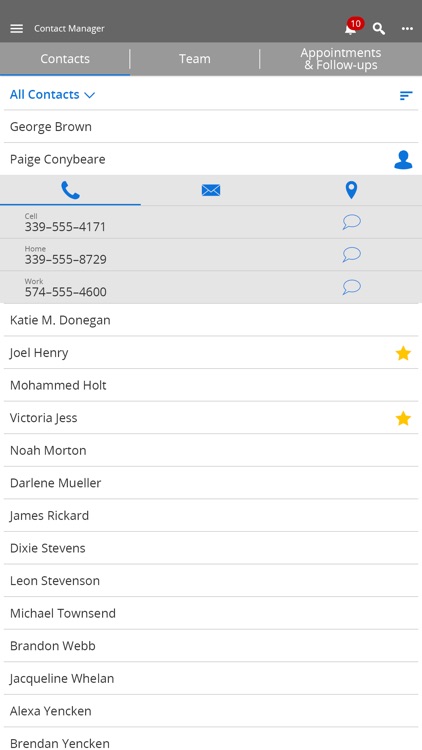The image appears to be a vertical screenshot of either a computer or cell phone interface, primarily featuring a white and black color scheme with gray highlights. At the top, there's a gray toolbar labeled "Contact Manager," accompanied by a notification bell icon with a red badge displaying the number 10. Below this, a lighter gray navigation bar contains options labeled "Contacts," "Team," "Appointments," and "Follow-ups," with "All Contacts" highlighted in blue, indicating it has been selected.

The interface includes phone, envelope, and pin symbols, followed by a list of phone numbers presented on a gray background. Beneath this section, over a white background, are vertically-separated names: KDM Donegan, Joel Henry (marked with a yellow star to the far right), Mohamed Holt, Victoria Jess (also marked with a yellow star), Noah Morton, Darlene Mueller, James Ricard, Dixie Stevens, Leon Stevenson, Michael Townsend, Brandon Webb, Jacqueline Whelan, Alexa Yechin, and Brendan Yechin. Each name is clearly delineated by lines.